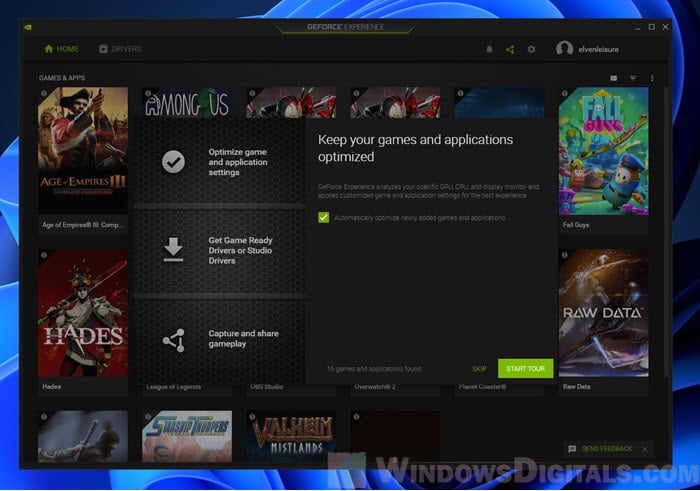This image is a computer screenshot displaying a user interface, likely from a gaming platform or optimization software. The background features a dark theme decorated with scattered blue circles, predominantly situated in the top right, bottom left, and bottom right corners. Centered on the screen is a large black rectangle showcasing a game website interface.

In the upper left corner of the interface, there is a home icon labeled "Home." On the far right, an account name is visible, indicating a logged-in user. Flanking the central content on both sides are images of various games. On the left side, the top image shows a pirate, identified as the game "Age of Empires." Below it is an image of a soldier wielding a large sword, representing the game "Hades." On the right side, the upper image features a green background with oval-shaped characters, indicating the game "Fall Guys." Beneath it, a gray background displays a character holding a sword, for the game "Raw Data."

Dominating the center of the screen, a message reads, "Keep your games and applications optimized." To the left of this message, there is a submenu with options including "Optimize game and application settings." Further down, additional options are listed: "Get Game Ready drivers" or "Studio drivers," and "Capture and share gameplay." The layout and features suggest a focus on maintaining and enhancing gaming experiences through optimized settings and updates.